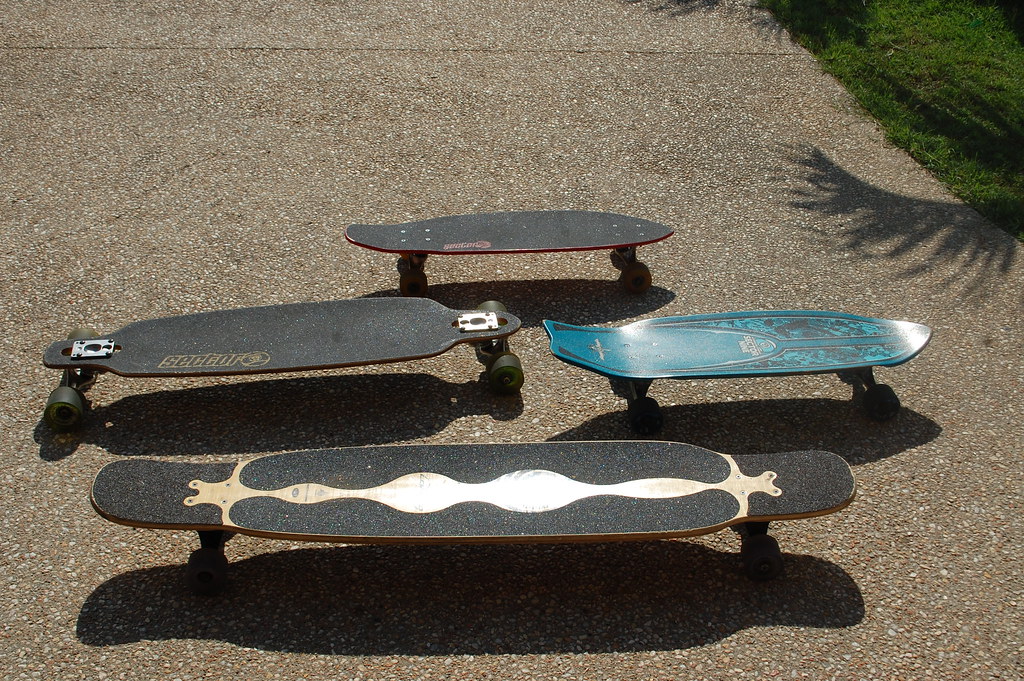The image showcases an outdoor photograph of four skateboards arranged horizontally on a textured, small-pebble light brown sidewalk, distinct from regular cement. The skateboards are on display in the foreground of the photograph. Starting from the top, the smallest skateboard is black with a traction top, resting with its wheels on the concrete. Moving to the center, there are two skateboards: one on the left, also black with a silver metal wheelbase, and another on the right featuring a teal color adorned with black markings. In the forefront, the longest skateboard is notable for its black surface with a striking white wavy design pattern down the middle. Additionally, in the upper right corner of the image, there is a hint of lush green shrubbery casting a shadow resembling a palm leaf onto the sidewalk, adding to the image's outdoor ambiance.